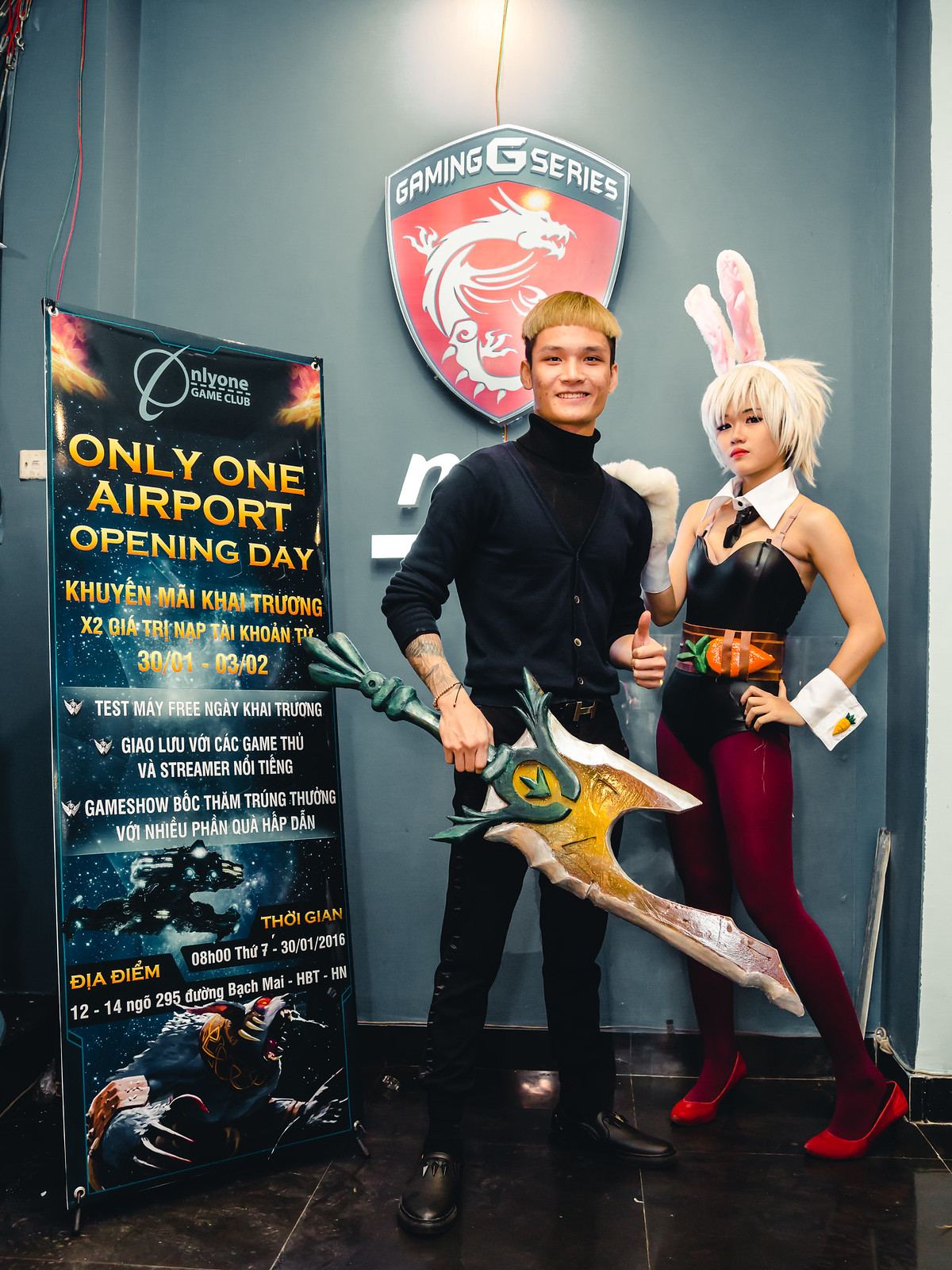This vertical rectangular image is a detailed photograph likely intended to advertise a product or event, characterized by vibrant colors and a dynamic setting. Positioned against a medium aqua wall depicting a red and white dragon crest labeled "Gaming G Series," the photograph features two young, Asian individuals in cosplay. The male, about 16 years old with blonde hair, dons a black turtleneck and trousers, and brandishes a large green and gold fantasy sword, giving a thumbs up with a smile. Beside him, a 15-year-old female with a white wig and bunny ears is dressed in a striking outfit comprising red pumps, dark red hose, a black leather bustier, and an orange-belted swimsuit displaying a carrot emblem. Her ensemble is completed with white cuffs and a collar with a little tie. On the left side of the image, a dark, action-themed poster with yellow text reads "Only One Airport Opening Day," and includes non-English text detailing the event's schedule. The setting also features a dark wooden floor adding contrast and depth to the scene.